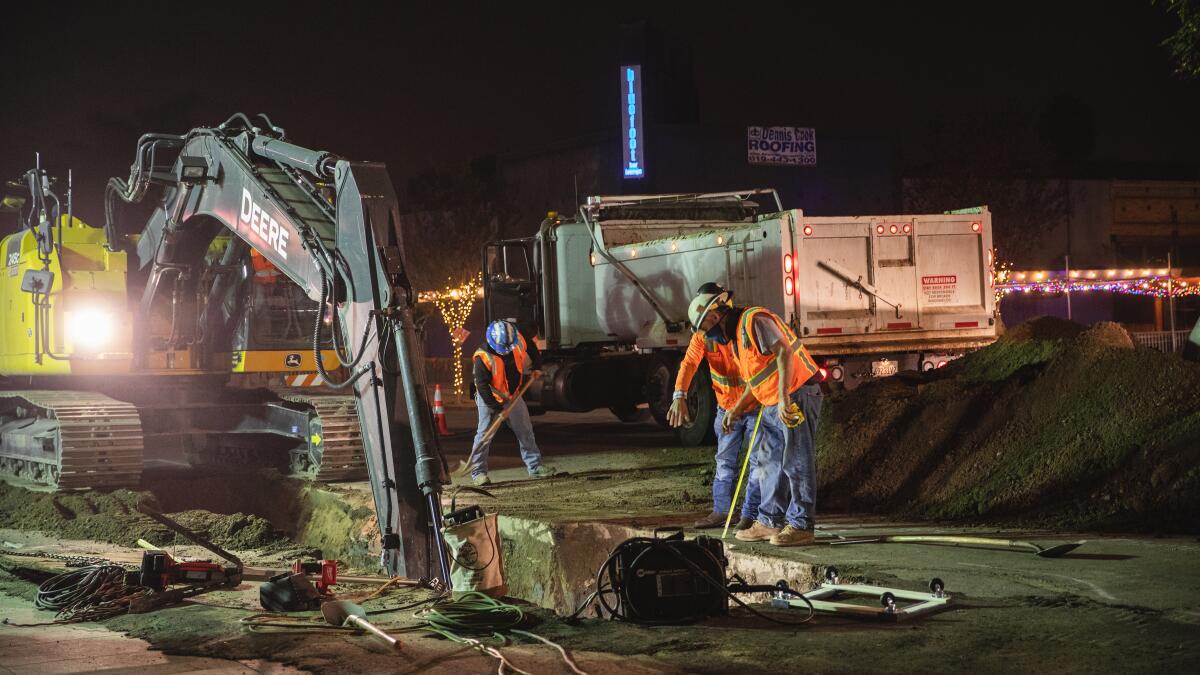In this detailed and realistic painting of a nighttime construction scene, three construction workers, all wearing orange safety vests, blue jeans, and boots, are busily engaged with their tasks around a large trench. On the left side of the image, a massive, yellow John Deere excavator with tank-like rollers is actively digging, its bucket hidden deep within the trench. The word "DEERE" is clearly visible on the excavator's arm. 

Surrounding the trench are various pieces of equipment and cables, and the bright headlights from a large utility truck illuminate the workers and their immediate vicinity. The worker at the forefront, distinguishable by his blue hard hat and black long-sleeved shirt, holds a broom-like tool, pushing dirt or debris. Near the center-right, another worker in a face mask watches the digging intently, while a second worker, partially obscured, stands behind him.

In the background, a string of lights hangs over the scene, and a sign reading "Dennis Cook Roofing" is visible on a building behind the workers, next to an illegible blue neon sign. The sky is an inky black, accentuating the intense focus of the workers below as they navigate the construction site, a dirt-covered terrain resembling a golf course.